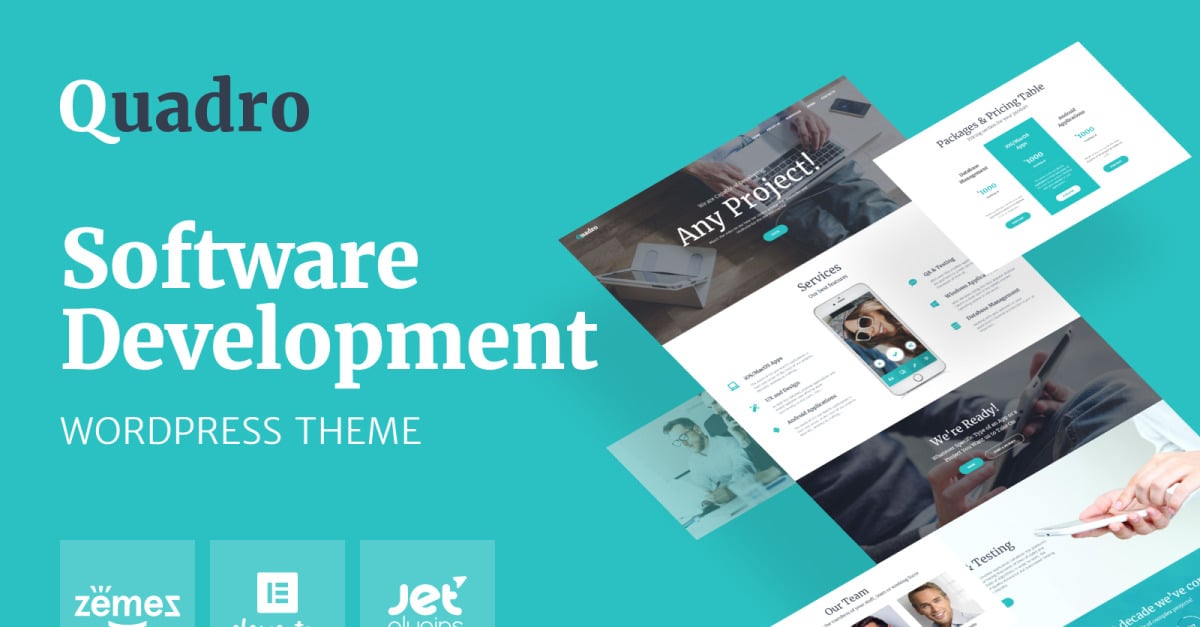An advertisement featuring a turquoise-colored background is prominently displayed. The focal point is the company name "Quadro," with a distinctive white "Q" and the rest of the letters in black. Most of the text in the ad is white. Below the company name, in large, bold text, are the words "Software Development." Underneath this, in a smaller and different font, the phrase "WordPress Theme" is written.

Three squares are beneath the main text, each containing some information. One square reads "Xemnas," the content in another is unreadable, and the last one appears to say "Jet Something."

On the right side of the ad, there is a graphic representation of an angled webpage layout, illustrating a template that utilizes the company's theme. This layout features text at the top indicating "Any Project," accompanied by a background image labeled "Services." In the center is a graphic of a phone, and there's additional text on both the left and right sides. The color scheme throughout the layout matches the ad’s overall design, utilizing white and turquoise tones.